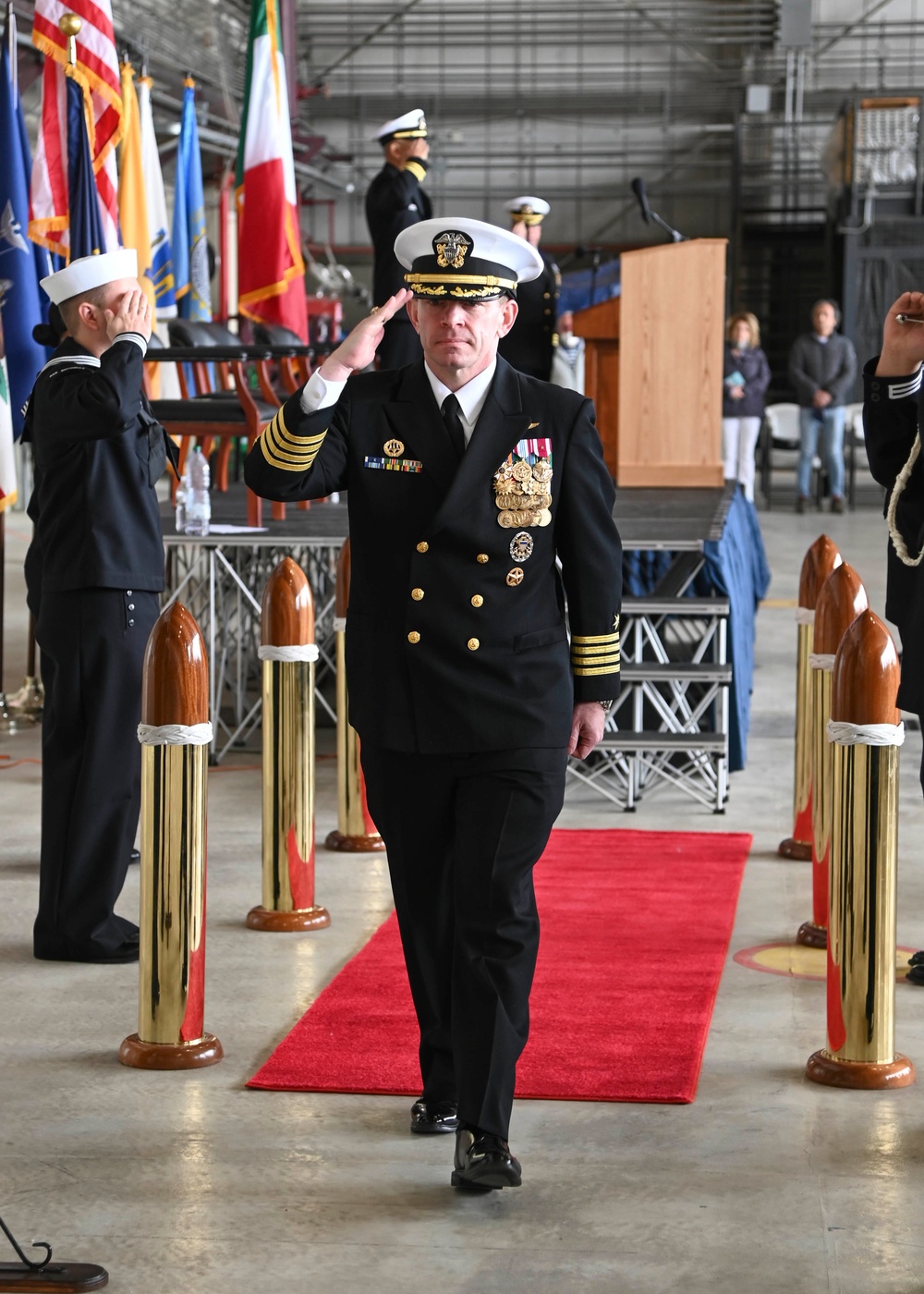The image captures a solemn military ceremony, with a central figure who appears to be a high-ranking officer, perhaps a commander or lieutenant. He is in full military uniform adorned with numerous medals, saluting someone out of the frame. The officer's attire includes a distinctive white hat, highlighting his prominence in the scene. Beside him stands another military personnel, possibly from the Navy, dressed in a dark blue uniform and a sailor-like white hat, though his front is not visible to reveal any medals.

In the background, a mix of military personnel and regular civilians can be seen. The military members stand on a stage, behind which a variety of flags are displayed, including the American flag and others from different countries. The scene is set against a bright color palette featuring red, blue, white, and gold hues, giving it a vivid and formal atmosphere. Civilians, easily identifiable in casual attire like jeans, observe the proceedings from further back.

The foreground features a red carpet, flanked by special barriers resembling large lipsticks with brown domes at the top, adding to the ceremonial ambiance. The image is in color and seems professionally taken, emphasizing the respect and significance of the event.